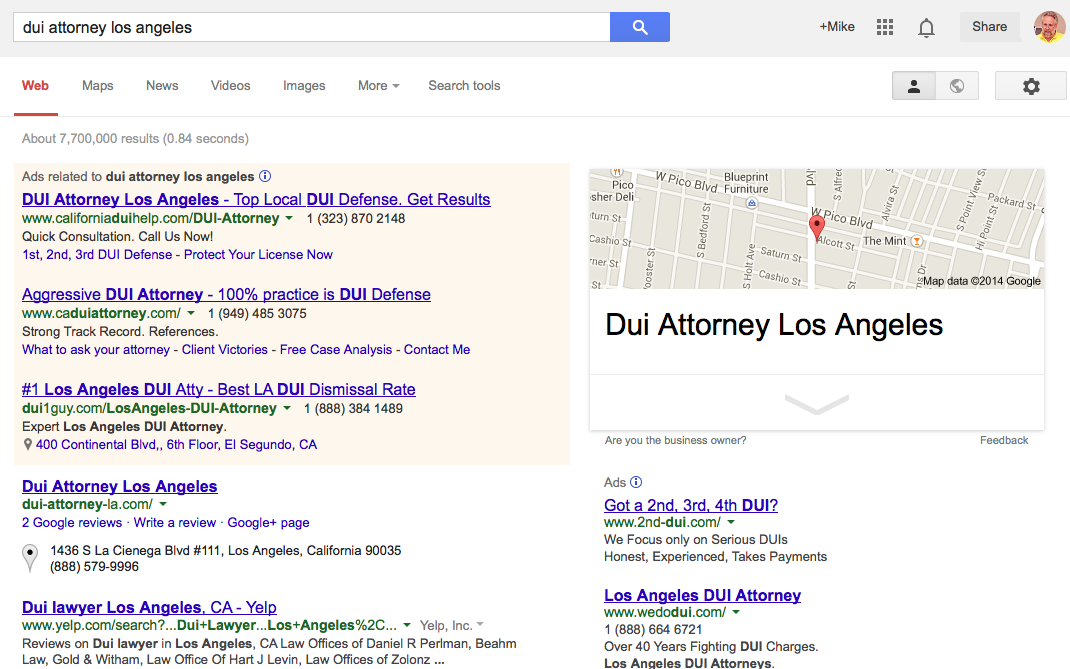This image depicts a user interface in landscape mode, showcasing a search engine results page (SERP) for the query "DUI attorney, Los Angeles." The upper portion of the screen features a search bar with the query entered, and the search button to its right. In the top right corner, there are additional options including a "+ Mike" icon, presumably representing the user's profile, along with a share button.

Below the search bar, there are various navigation options such as "Web," "Maps," "News," "Videos," "Images," "More," and "Search tools." "Web" is highlighted in red and underlined, indicating the selected category, followed by a display of approximately 7,700,000 results. The page is divided into multiple sections: a cream-colored section at the top contains ads related to "DUI attorney, Los Angeles," featuring terms such as "Aggressive DUI attorney," "#1 Los Angeles DUI attorney."

Beneath the ads, there is a white section showing organic search results for "DUI attorney, Los Angeles" and "DUI lawyer, Los Angeles." Towards the upper right-hand side of this section, a map is displayed pinpointing a DUI attorney located on Alcott Street. Additional advertisements for DUI attorneys in Los Angeles are listed below, including links and descriptions for specific legal services, such as handling second, third, and fourth DUI offences. These links are designed to direct users to different law office websites specializing in DUI defense cases.